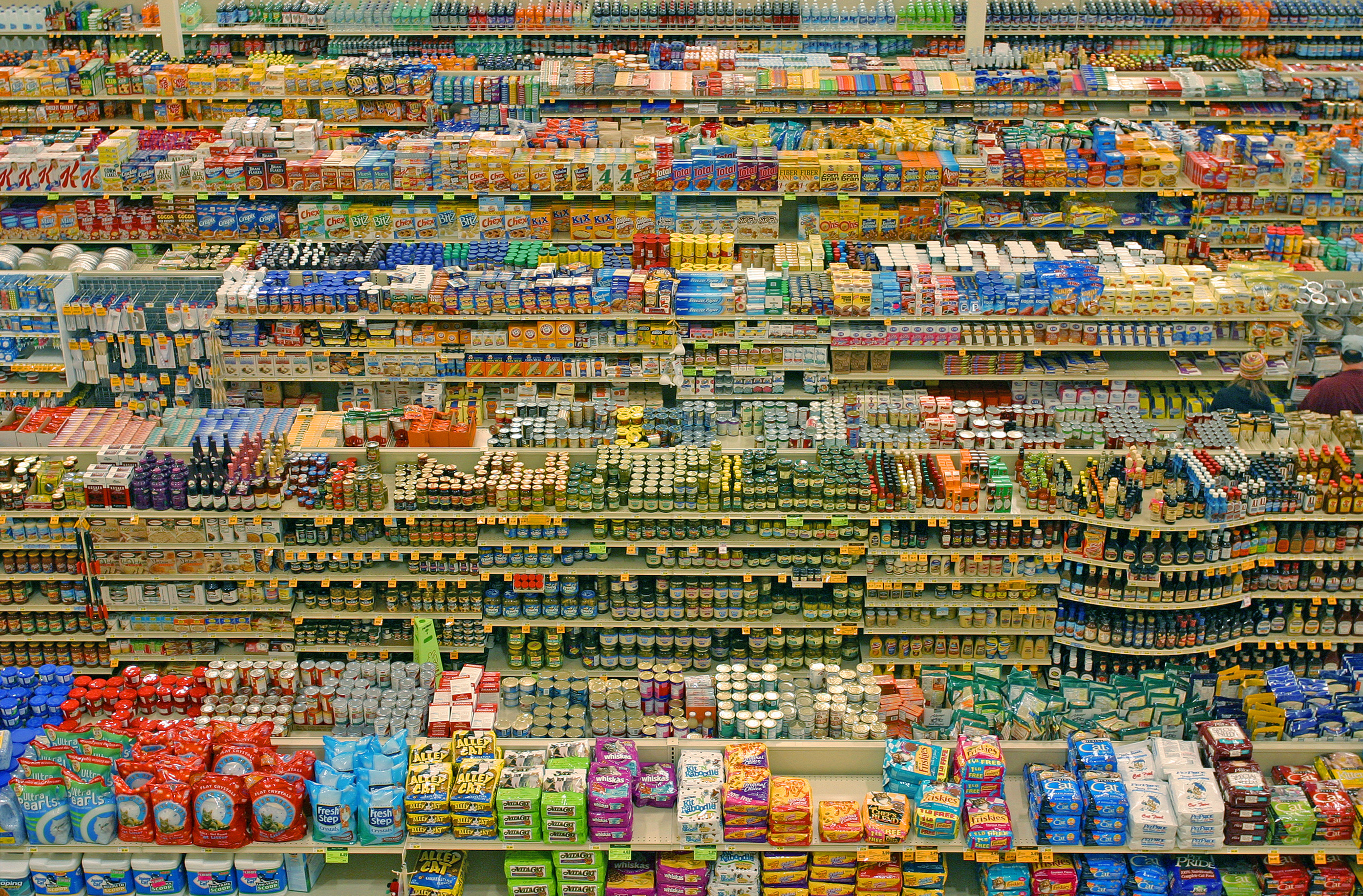A high-angle shot captures the vast interior of a large supermarket, showcasing a detailed view from near the ceiling. The image reveals expansive rows of fully stocked shelves, each brimming with an array of products. From this vantage point, it's clear that the store offers a broad spectrum of items, though the specifics are indiscernible due to the distance. The shelves display a multitude of items in bags, boxes, and bottles, featuring a diverse palette dominated by blue and yellow hues. The layout suggests sections dedicated to household cleaning supplies and another to medications and supplements. Towards the back of the store, a section with bottled sodas is faintly visible. Interestingly, the entire scene unfolds devoid of any shoppers, emphasizing the abundant inventory available—even more than one might ever use in a lifetime.